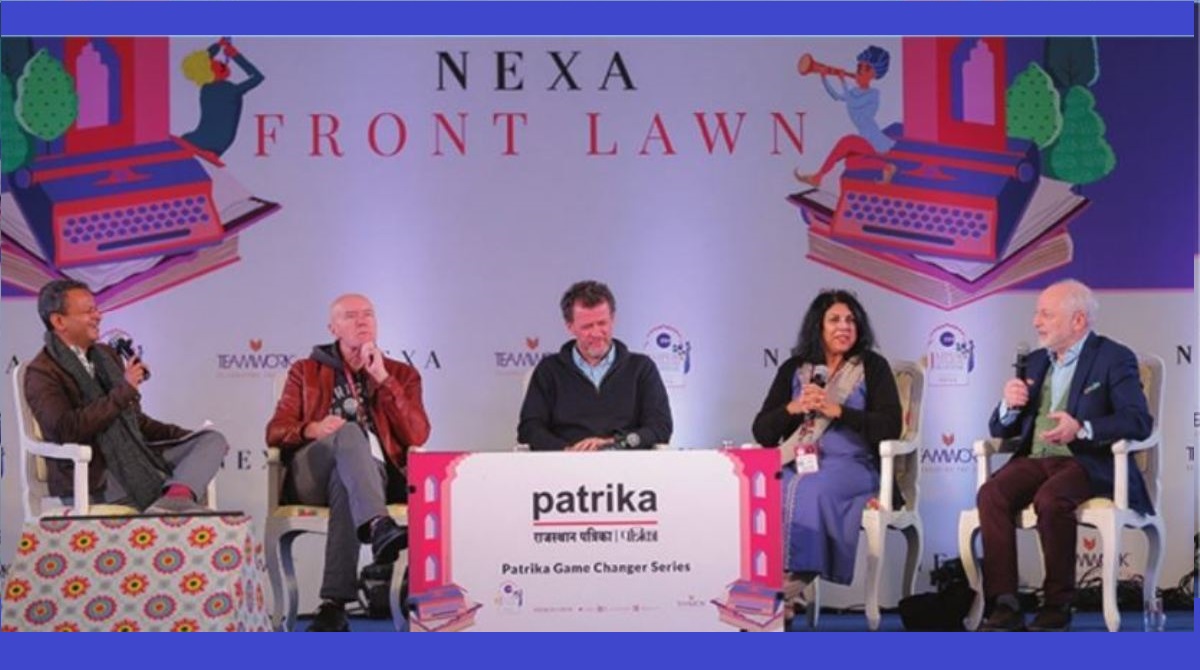The image depicts a stage setting, likely at a conference, featuring five older individuals seated in a round table format. Behind them is a white wall adorned with illustrations of cartoon people, giving the backdrop a lively feel. The wall prominently displays the text "Nexa" in black and "Front Lawn" in red, with further decorative elements including a typewriter on a stack of books from which a person seems to be emerging, holding binoculars, and another figure wearing a blue dress playing a trumpet—all set against what appears to be a Middle Eastern architectural background.

The people on stage are each holding microphones, suggesting they are preparing to speak or are part of a panel discussion. From left to right:
- The first man is brown-skinned, wearing a suit.
- Next to him is an older, bald, Caucasian man in a red jacket and gray pants.
- The central figure is a man with brown hair, dressed in a black sweater, seated behind a white desk with pink borders. The desk prominently features the text "Patrika" and "Patrika Game Changer Series" on the front.
- The only woman on the panel is seated next to the central man, wearing a black sweater over a purple dress, with dark hair.
- The man on the far right has white hair, is older, and is dressed in a blue jacket and brown pants. 

The setting is bordered at the top and bottom by a thin blue rectangular border, adding a formal touch to the stage appearance.